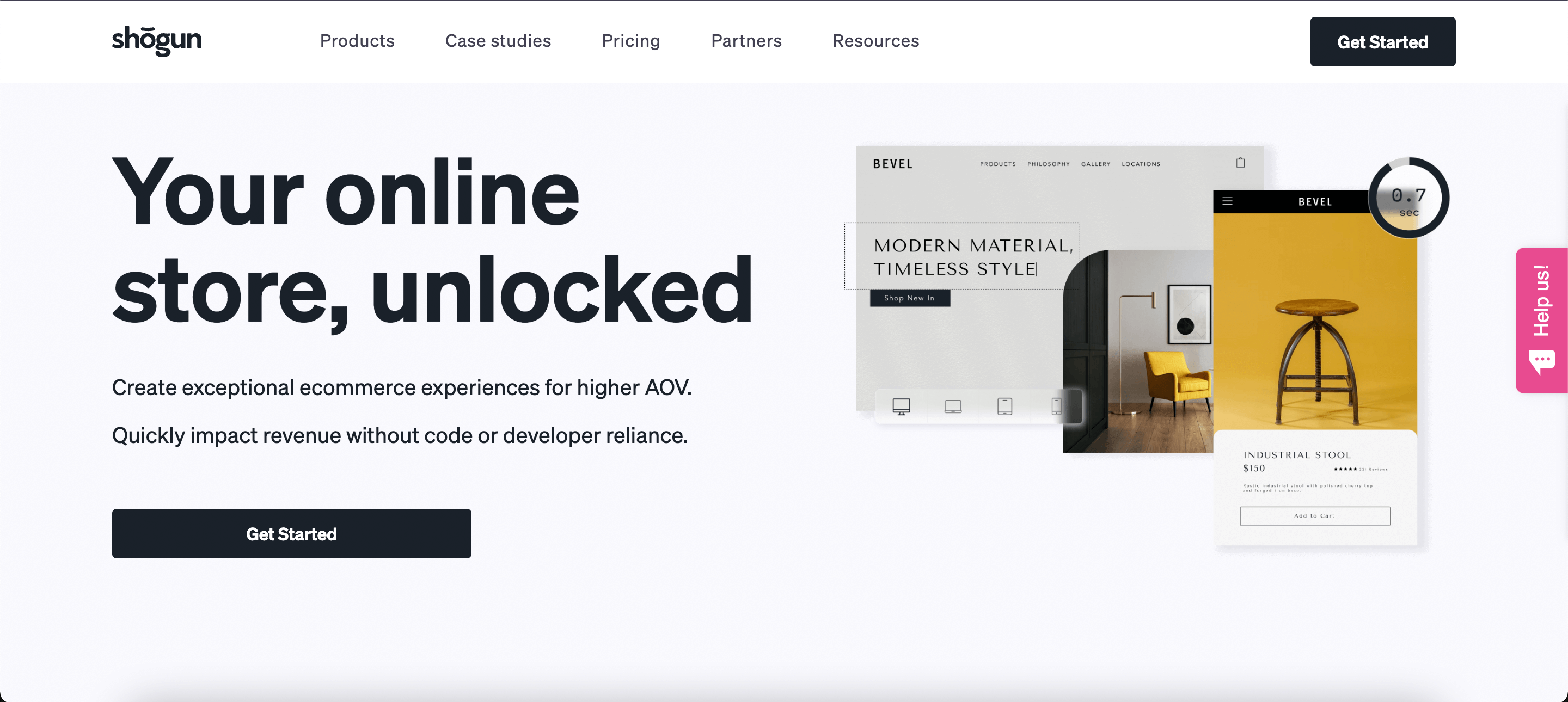The image is a detailed screenshot of the splash page for Shogun, a platform aimed at improving e-commerce experiences. Positioned in the top left corner is the Shogun logo, with a navigation bar featuring the links: Products, Case Studies, Pricing, Partners, and Resources. On the far right, there is a prominent black button labeled "Get Started" in white text.

The central tagline of the page reads, "Your online store unlocked. Create exceptional e-commerce experiences for higher AOV. Quickly impact revenue without code or developer reliance." Below this tagline, another black rectangular button also urges users to "Get Started," again in white text.

To the right of the main text, there is an image showcasing a sample web page named "Bevel." The sample features navigation options including Products, Philosophy, Gallery, and Locations. Below the navigation bar, there is a highlighted box titled "Modern Material, Timeless Style, Shop New In." This suggests that Bevel is a furniture store, as evidenced by the image of a stylish yellow chair placed in a living room setting, complete with a black wall on the right and a gray wall in the background.

In front of the chair, there is a depiction of a mobile screen showing an industrial stool priced at $150, characterized by a shiny, light-brown, round top and four arched legs. Accompanying this mobile screen image is a small circular indicator reading "0.7 seconds," potentially signifying the swift load time for the product display.

This screenshot emphasizes Shogun's core function in assisting users to enhance their e-commerce platforms by offering visually appealing and functional website elements, thereby optimizing user engagement and driving sales.